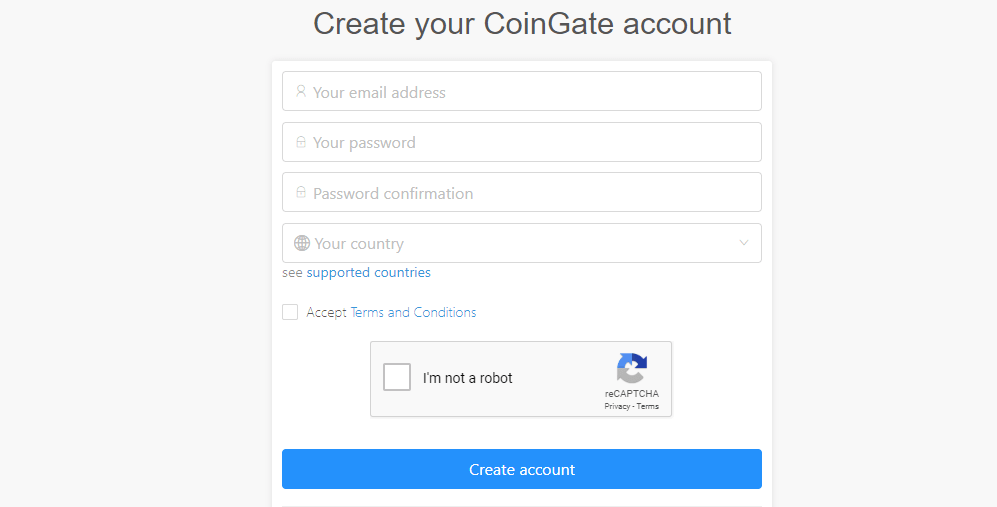The image displays the account creation page for a CoinGate account, as seen on a website. At the top of the page, there is a prominent header that reads "Create Your CoinGate Account." Below this header, there are four input fields arranged vertically. The first field is for entering an email address, followed by a field for creating a password. The third field requires password confirmation, and the fourth field is a dropdown menu for selecting your country of residence.

To the left underneath these fields, there is a clickable text labeled "See Supported Countries" in blue font, providing a link to view a list of countries supported by CoinGate. Below this, there is a checkbox labeled "Accept Terms and Conditions," with the terms themselves also highlighted in blue, indicating another clickable link.

Beneath these elements, there is a reCAPTCHA verification box with the statement "I'm not a robot," which users can click to confirm they are human. Finally, at the bottom of the page, there is a prominent "Create Account" button written in white text against a blue background.